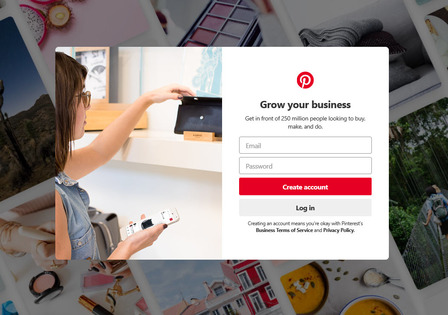The image is a promotional post from Pinterest showcasing a business growth opportunity. The background consists of various photographs placed on what appears to be a table. These photos depict scenes of nature, food, makeup, homes, and a pop-up box. 

In the foreground, there is an image of a young woman with brown hair. She is holding a smartphone in her right hand and has a gray pocketbook over her shoulder. She is dressed in a dungaree vest. Her left hand is interacting with a tablet that rests on what looks like a shelf, possibly within a retail store, suggesting she is considering a purchase.

To the right of this scene is the Pinterest logo, under which the text "Grow your business. Get in front of 250 million people looking to buy, make, and do" is displayed. Below this message, there are fields for entering an email address and password, followed by a red "Create Account" button and a gray "Log in" button. There is also some small print concerning services and policies, though it is difficult to make out clearly.